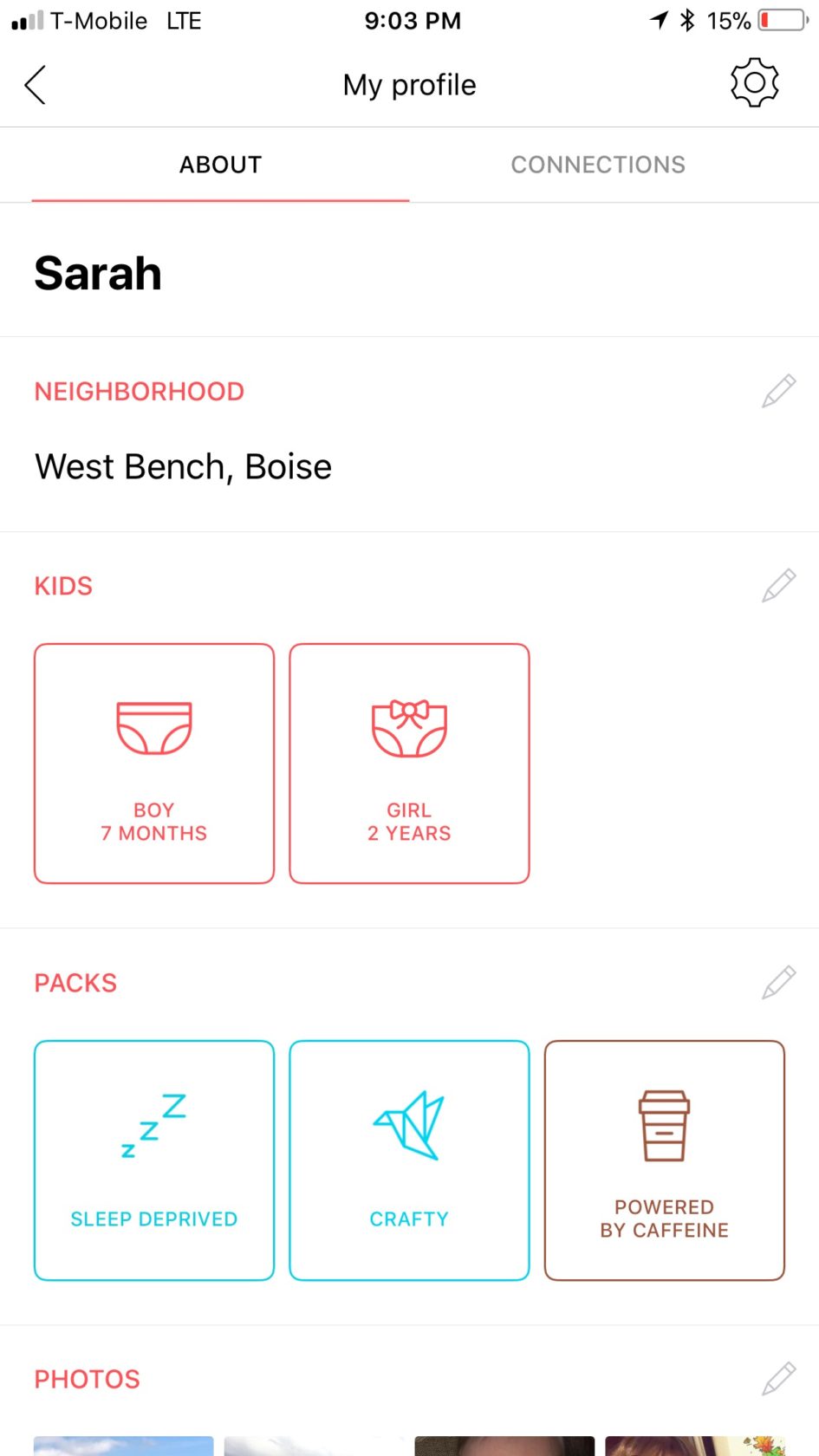The screenshot showcases a mobile phone interface with several elements prominently displayed. At the top, the phone shows a T-Mobile LTE signal with two bars, the current time noted as 9:03 p.m., and indicators for Bluetooth and location services being active. The battery icon displays a concerning 15% charge remaining.

Directly below this status bar, the interface presents the user's profile section, marked as "Sarah." Beneath Sarah's name, her neighborhood is listed as West Bench, Boise. Further details include a section labeled "kids," with icons representing a boy aged seven months, symbolized by a classic pair of white underwear, and a girl, similarly represented but differentiated by a small decorative bow.

Next, the "packs" subsection lists various statuses: "deprived" and "crafty" in green, suggesting some form of positive status, and "powered by caffeine" in brown, possibly indicating a humorous or casual note about energy levels.

At the bottom of the screen, there is a section titled "photos," displaying a narrow strip of five thumbnail images. Due to the limited size of these thumbnails, the specific content of the photos cannot be determined.